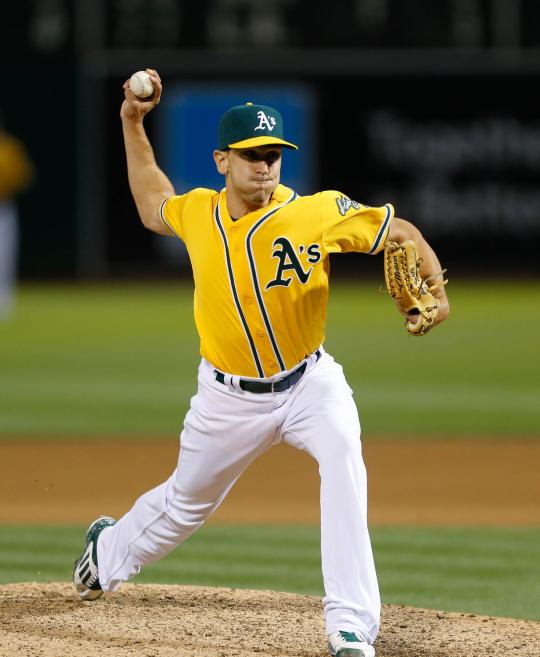The image is a detailed close-up of a pitcher from the Oakland A's on the pitcher's mound, dressed in a vivid yellow uniform top with a button-down design, accented by a dark A's logo on his left chest. His white pants are complemented by a black belt, and he's wearing a green cap with a yellow brim, bearing the team's emblem in white at the center. The photo captures him mid-pitch: his left foot is firmly planted on the gray and black mound, while his right foot and arm are extended backward, creating a dynamic pose. The pitcher's left hand, holding a mitt, is bent at the wrist with the glove facing up, and his right hand clutches a baseball behind him, poised to throw. His face reflects intense concentration, with closed lips and puffed cheeks, partially shadowed by the brim of his cap. The backdrop, although blurry, reveals the distinct layers of the baseball field – from the infield’s dirt and grass to the outfield wall, all set under the outdoor sky.